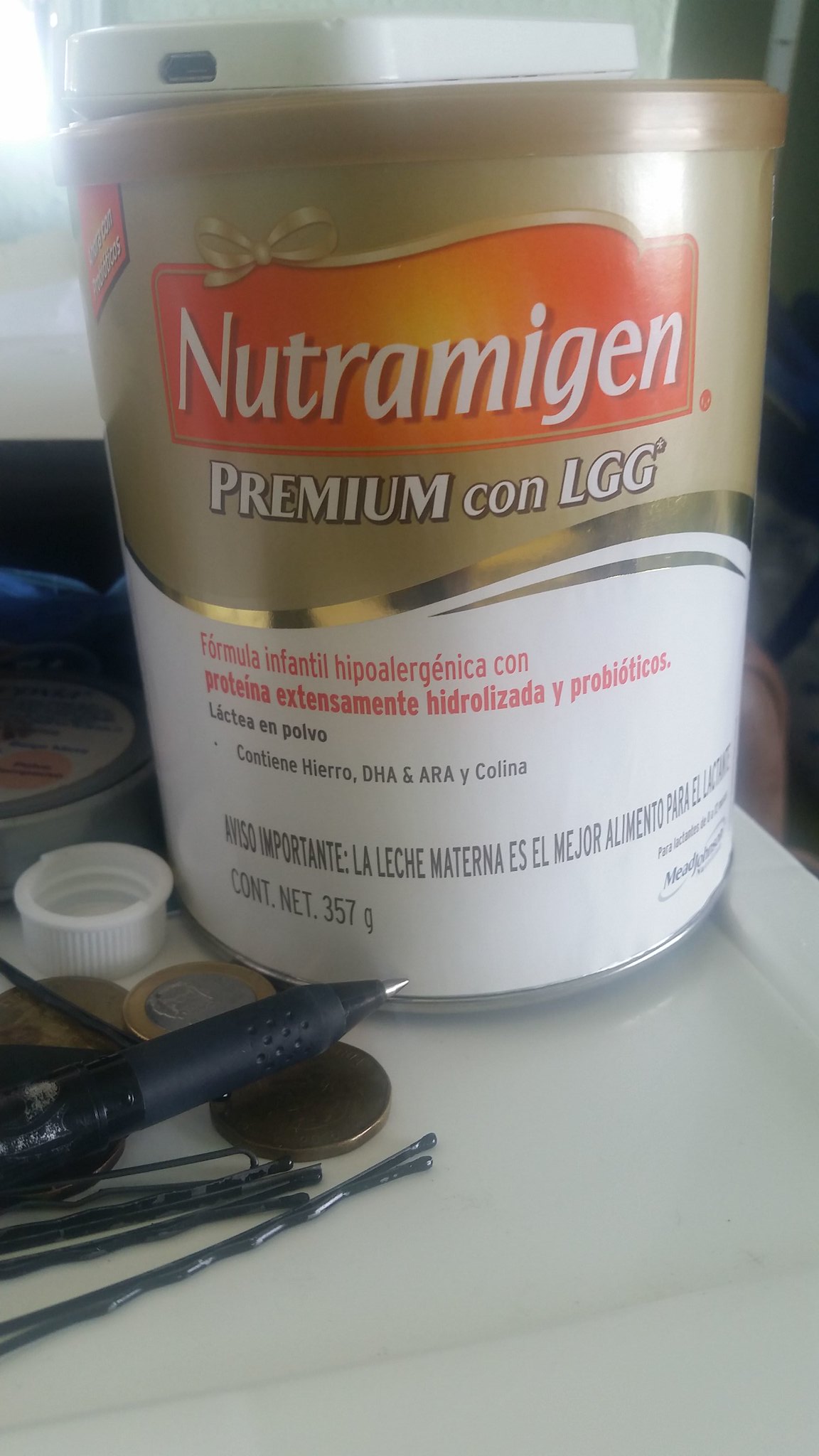A photograph showcases a Nutramigen can resting atop a pristine white table. The can features a gold lid and an orange banner emblazoned with the brand name "Nutramigen," spelled out as N-U-T-R-A-M-I-G-E-N. Below the banner, set against the gold, is the text "Premium Con L-G-G," followed by "Formula Infantile Hypoallergenica Con" and additional small print detailing the product's specifications. The bottom of the can clearly displays its net weight of 357 grams. Positioned to the left of the can are several loose items: a white bottle cap, a pen, a few bobby pins, and a couple of coins. The scene is illuminated by a light source coming from the upper left corner, casting soft shadows and highlighting the textures and details of the objects.